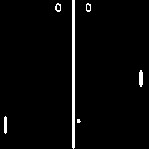The image portrays a classic arcade game, Pong, displayed in black and white on a small, approximately 1.5-inch square screen. The screen features a simple layout with a thick white line dividing the two black halves, representing the net. Each side of the screen has a vertical white paddle; the left paddle is positioned towards the bottom, while the right paddle is situated more centrally. At the top of the screen, the score is shown as 0-0, indicating the game has just started. A white ball is depicted crossing the middle court, appearing to have just bounced off the right paddle. The image, evocative of the original Pong game, shows noticeable pixelation, underscoring its vintage quality and simplistic graphics. The overall small size and basic design suggest it might be an image captured on or intended for a mobile phone screen.